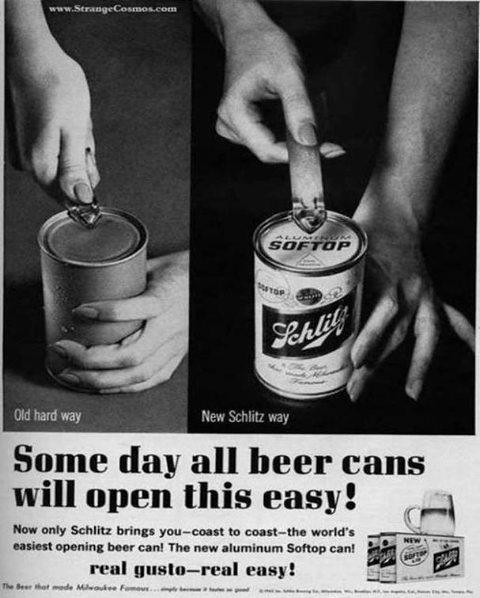This vintage beer advertisement, likely from the 1950s or 1960s, features two black-and-white images side by side. On the left, the image depicts hands using an old-fashioned can opener to puncture an unlabeled tin can, emphasizing the "old hard way" of opening cans. Beside it, on the right, a woman's hands are shown effortlessly opening a can of Schlitz beer with a modern opener, showcasing the "new Schlitz way." The Schlitz can prominently displays a "soft top" label, highlighting the ease of opening attributed to the new aluminum design. The bottom of the ad reads, "Someday all beer cans will open this easy. Now only Schlitz brings you coast to coast the world's easiest opening beer can, the new aluminum soft top can. Real gusto, real easy." Additionally, there's a small icon depicting a case of Schlitz beer, reinforcing the brand's innovative packaging.